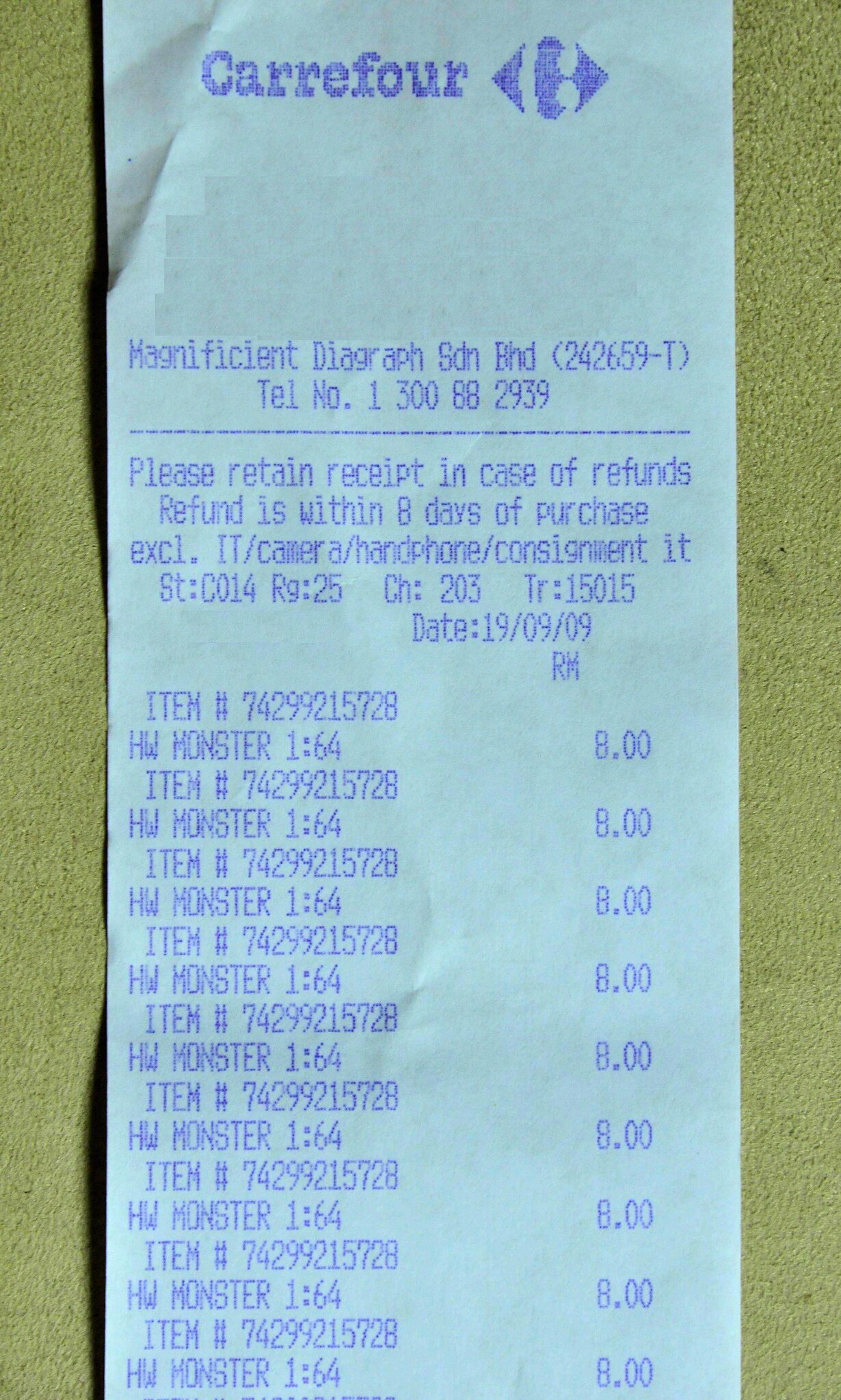The image shows a close-up photograph of a receipt from Carrefour, a supermarket, lying flat against a greenish-yellow background with a textured, almost spongy appearance. The white receipt, bearing blue text, has the store name "CARREFOUR" at the top, accompanied by its logo featuring two opposing triangles with a blue area in the center. Below that, the text includes the store’s address "Magnificent Diagraph, S-D-N-B-H-D, 242659-T" and the telephone number "1-388-2939."

Further down, there's a notice stating "Please retain receipt in case of refunds. Refund is within eight days of purchase," with exclusions outlined for IT camera handphone consignment items. The receipt is dated "19/09/09."

The main section of the receipt itemizes a single product repeated nine times: "H.W. Monster," priced at 1.64 each and totaling 8.00. The receipt's text and structure are partially cut off at the bottom of the image, indicating the photo does not capture the entire document.